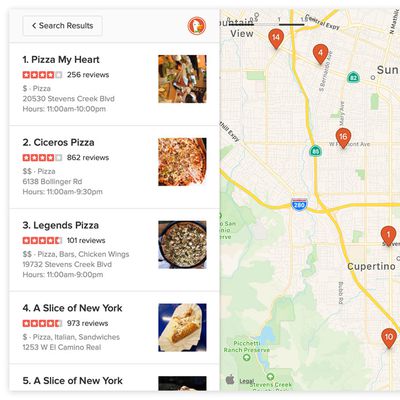**Detailed Image Caption:**

The image appears to be a screenshot captured from DuckDuckGo's interface, showcasing search results for pizza places. The overall layout includes a white background with a smaller white box on the left-hand side, featuring a right-pointing arrow labeled "Search Results" in black text. Adjacent to this is the DuckDuckGo logo, which is a red circle containing a white duck with a yellow bill facing right.

The search results list five pizza places, detailed as follows:

1. **Pizza My Heart**: This establishment has 256 reviews, accompanied by an icon of a pizza slice.
2. **Ciro's Pizza**: Rated with four stars from 862 reviews, also represented by a pizza slice icon on the right.
3. **Legend's Pizza**: Boasts four and a half stars out of 101 reviews, depicted with a larger pizza icon.
4. **Slice of New York**: Holding a high rating of four and a half stars with 973 reviews, this place too uses a pizza slice icon.
5. **Slice of Pizza**: The details for this listing are partially cut off, obscuring the number of stars, reviews, and the pizza slice icon.

On the right side of the image is an Apple Maps interface, distinguishable by the small gray Apple logo at the bottom left corner. The map features a creamish white tone for buildings, a white color for main streets, a lighter yellow for side streets, and green areas representing parks. The map also includes numerical indicators positioning the pizza places within the mapped area.